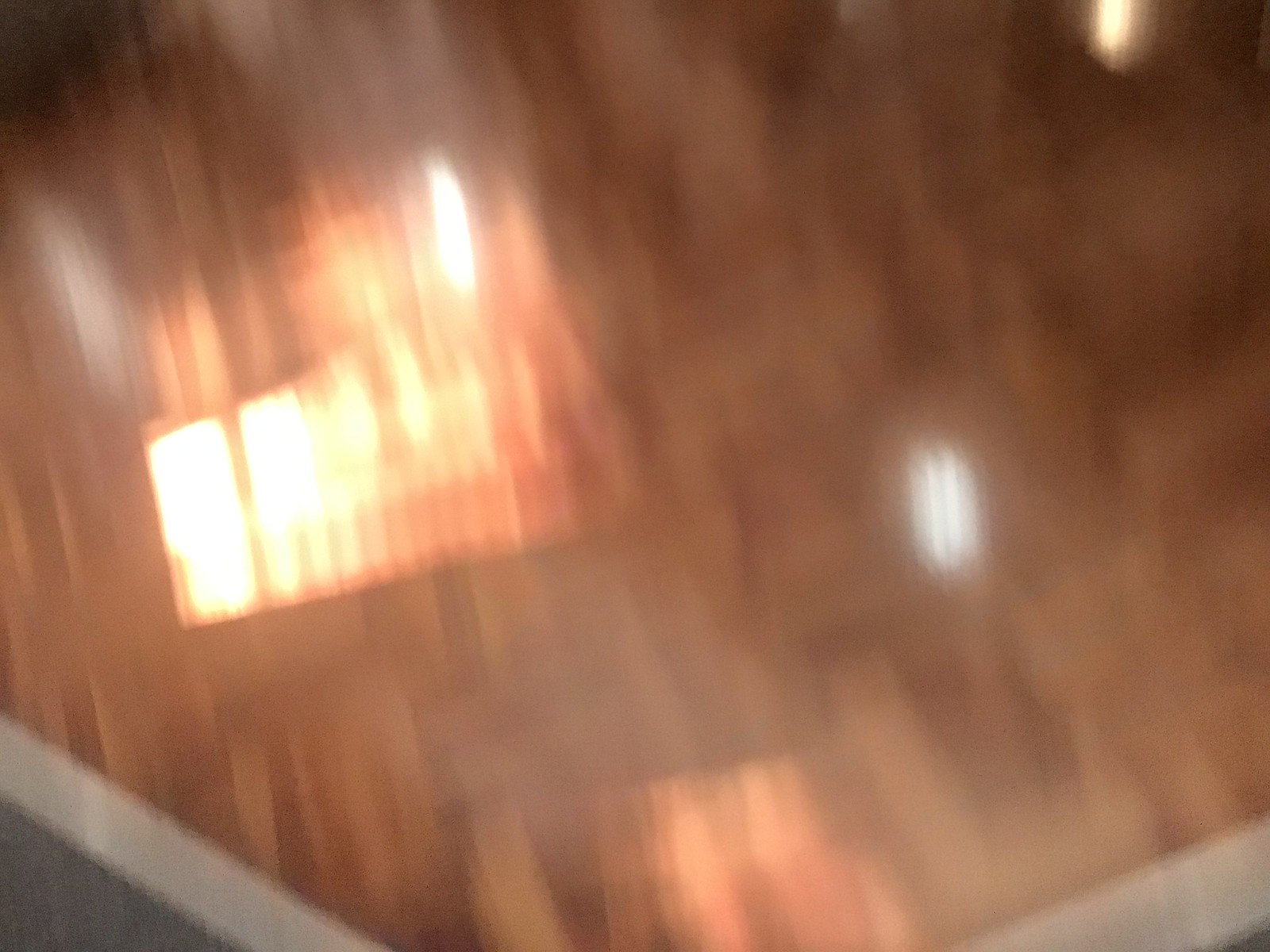The photograph is notably low in quality and extremely blurry, making it challenging to identify the subject matter. Captured out of a window—possibly from a building or a vehicle—the image features a small section of a border in the bottom-left corner, potentially indicating part of a wall or window frame. In the distance, several lights are visible, appearing rectangular and likely belonging to a sign or an illuminated LED billboard, glowing in shades of yellow and orange. Additional lights can be seen further away, perhaps suggesting distant headlights. The significant vertical motion blur suggests the camera was shaking considerably at the time the photo was taken, rendering the overall scene nearly indiscernible.